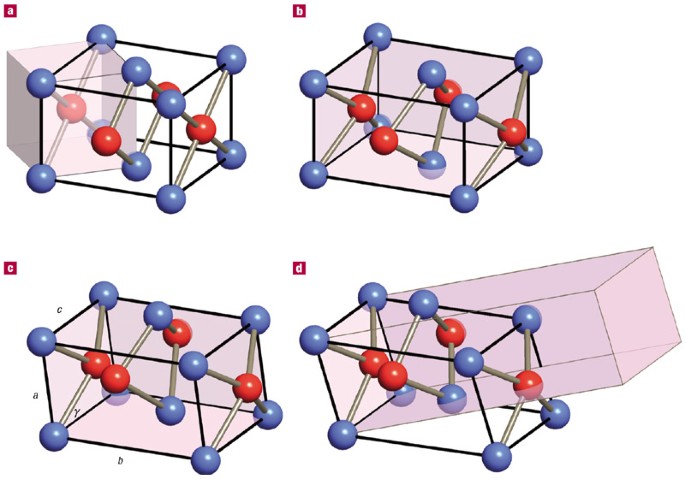This image features four scientific diagrams labeled A, B, C, and D, arranged in a 2x2 grid with A and B on the top row and C and D on the bottom row. Each diagram showcases a 3D model consisting of blue balls connected by black lines and red balls centrally located within a cubic structure made by white sticks. 

In Diagram A, the blue balls form a clear cubic structure with red balls positioned centrally. Diagram B similarly features a cubic arrangement, but the structure appears slightly larger, and the red balls are shifted compared to A. 

Diagram C continues the trend with the blue balls forming a cube, but noteworthy changes in the positions of both blue and red balls indicate an ongoing process. Finally, in Diagram D, the cube formed by blue balls appears more complex and larger, with some red balls extending beyond the structure, suggesting a significant transformation from the initial configuration.

Overall, the sequence from A to D illustrates a dynamic process involving blue and red balls connected by lines and sticks, indicating shifts and changes within a 3D molecular or atomic framework. The exact scientific context remains unclear without further information.